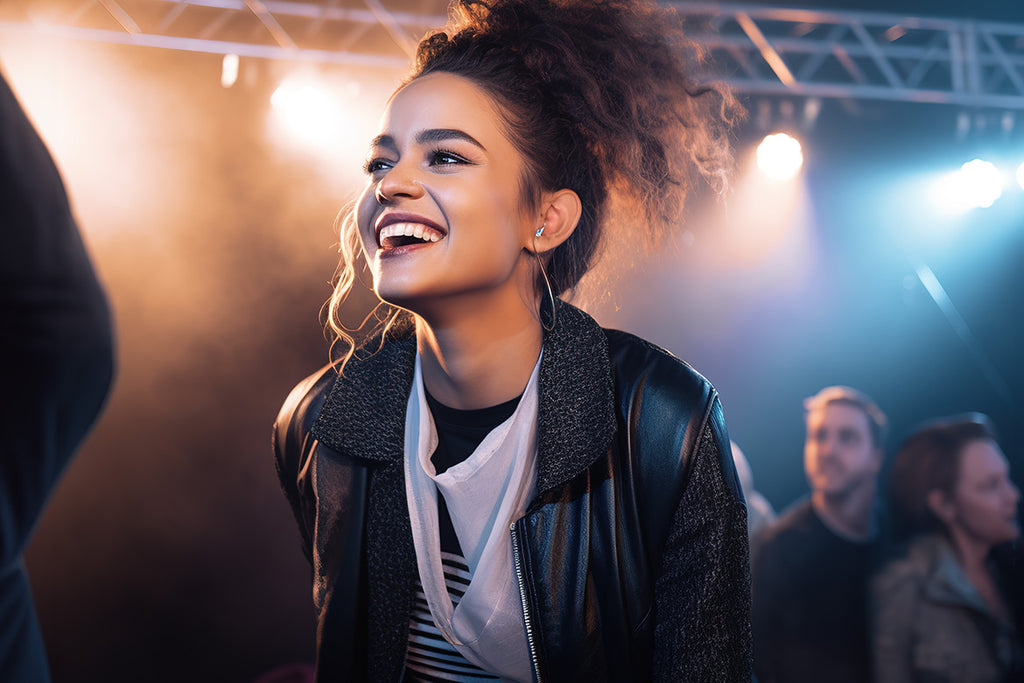In this vibrant photograph, a young woman of color is captured as the focal point, her joyful smile radiating under the bright stage lights. With her curly hair pulled into a top bun and earbuds in her ears, she exudes excitement and happiness. She is dressed in a dark leather jacket with an attached fur collar, layered over a white blouse and a black-and-white striped shirt. Her neatly defined eyebrows and broad smile reveal a sense of utter joy and amazement, likely at a concert or a lively club. The background features blurred attendees, adding depth while ensuring the woman's exuberant expression remains central. Blue and yellow lights, hanging from scaffolding and surrounded by fog, illuminate her from both sides, with the yellow light being more prominent. This lighting effect enhances the festive atmosphere of the scene, encapsulating a moment of euphoria and music.